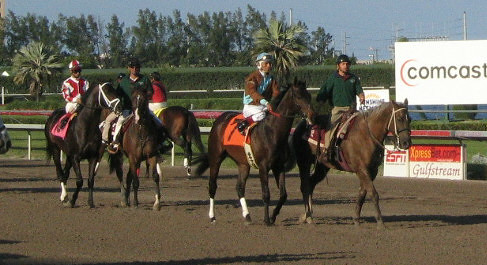The image depicts a horse race at a track under a clear blue sky. In the foreground, there are five dark brown horses being ridden by jockeys. Four horses are moving to the right, with one horse heading away from the camera. The jockeys, all men, are dressed in distinctive colorful outfits and helmets: one in red and white, one in light brown pants with a dark green top and dark blue hat, one in dark brown top with light white trousers, and another in a dark green jersey. The ground of the track is a dark brown, possibly muddy, surface. The background features neatly shaped green bushes, trees, and metal rails adorned with advertisements. Visible signs include prominent ones from Comcast, Gulfstream, and an "Express" sign above the Gulfstream advertisement. The scene is lively and dynamic, capturing the essence of a competitive horse race.